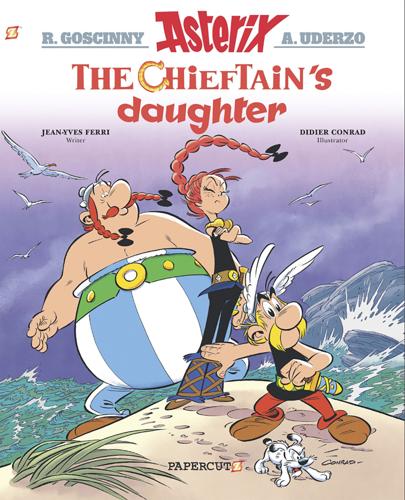This detailed cover illustration of "The Chieftain's Daughter," by R. Gosinny and A. Uderzo, features a vibrant cartoon scene with multiple characters and a dynamic backdrop. The title is prominently displayed at the top in bold red asterisks for emphasis. Beneath, in gray lettering, it credits the authors "R. Gosinny" and "A. Uderzo," and mentions Jean-Yves Ferry on the left and Didier Conrad on the right. The background showcases a tumultuous ocean with crashing blue waves under a purple sky, dotted with flying seagulls. Centered in the foreground are three distinct characters: a large, obese man with a red mustache and braided hair, wearing blue and white striped pants; a slender girl with long, swinging red braids, clothed in a black top and pants with intricately colored boots; and a shorter man donned in a black sleeveless shirt, red pants, and brown shoes. Accompanying them is a small white and black dog. The image's lively composition and colorful details hint at an adventurous story, blending elements of whimsy and excitement.